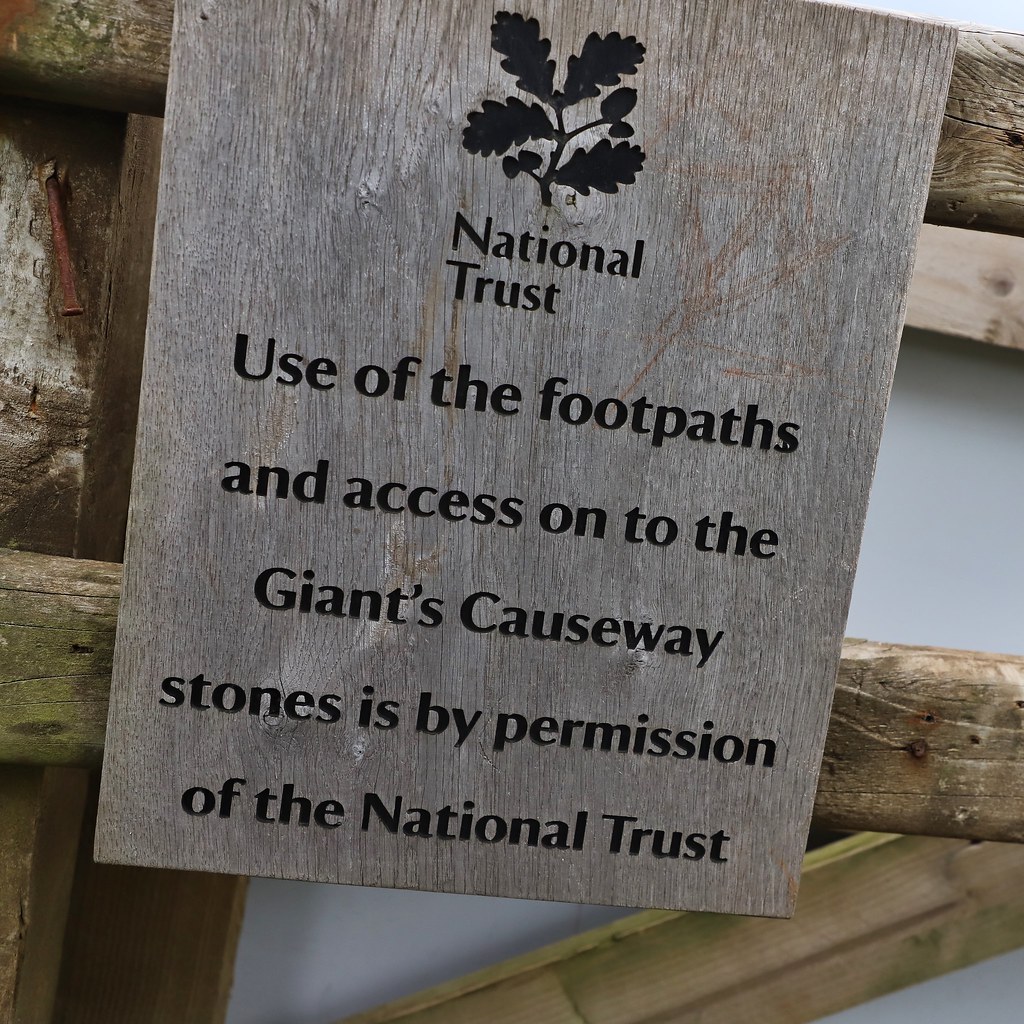The image depicts a rustic, weathered wooden sign nailed to a lighter wooden fence or barrier, possibly outdoors. The sign prominently features a logo at the top, consisting of a graphic of oak leaves and acorns, indicative of the National Trust. Below the logo, the sign reads in black print: "National Trust. Use of the footpaths and access onto the Giant's Causeway stones is by permission of the National Trust." The old-fashioned nails and worn texture of the sign add to its historical ambiance, suggesting it is a point of interest for tourists, possibly highlighting the importance of preserving heritage sites. Two horizontal wooden planks frame the sign in the photograph, providing context and dimension to the scene.